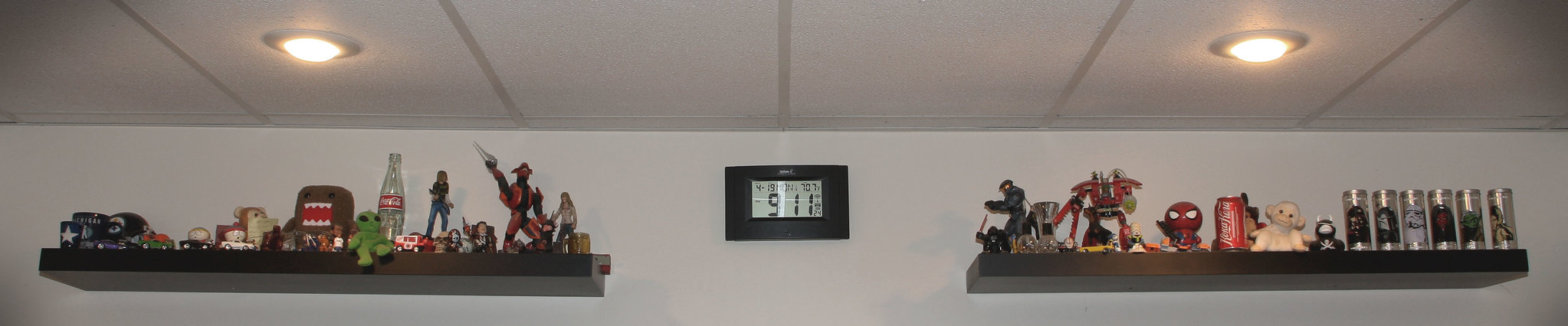The photo is a long, narrow rectangle, primarily showcasing an indoor scene. The top section of the image features a ceiling segmented into rectangular panels, adorned with two circular light fixtures. Positioned centrally on the wall below the ceiling is a black rectangular thermostat reading 91°F. Flanking the thermostat, there are two brown wooden shelves. 

On the left shelf sits a collection of vintage items, including an old Coca-Cola bottle and several action figures. The right shelf holds a variety of collectibles, including what appears to be a transformer figure, old collectible glasses or cans with images on their fronts, a Coca-Cola can, a miniature Spider-Man figure, and a doll characterized by its large ears.